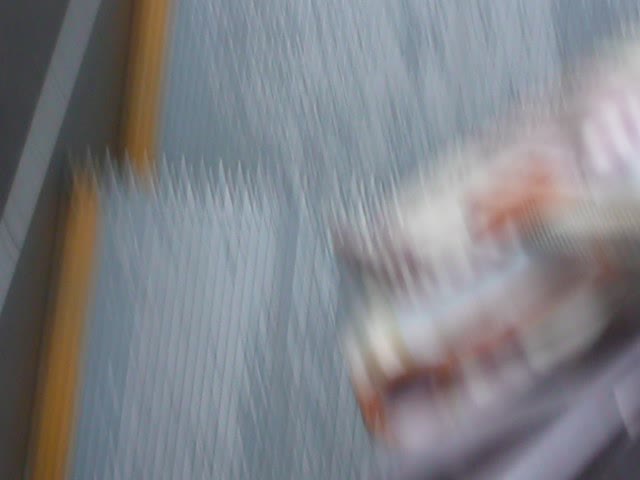This blurry photograph is challenging to interpret due to significant motion blur. However, a discernible white line streaks diagonally across the top left corner on a gray surface. The central area of the image appears to feature gray-colored, plastic sheet-like structures. On the right side, there's a suggestion of a bag, potentially purple in color with hints of orange details. The overall motion blur adds an element of ambiguity, making the exact contents difficult to identify with certainty.